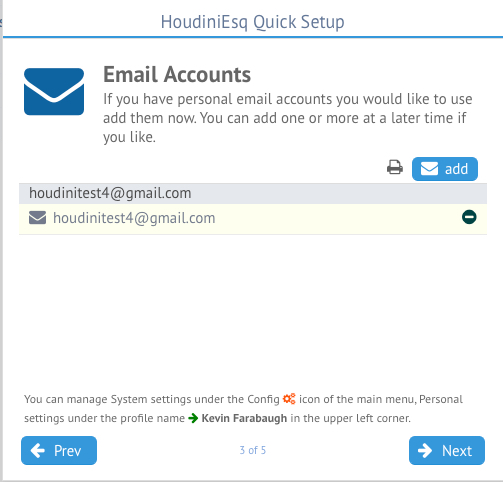This image depicts a section of an email website, specifically within the settings region, showing the left and bottom borders but not the top or right. At the top of the image, "Houdini Esquire" is prominently displayed. Below this, there's a header labeled "Quick Setup" followed by a blue separator line.

Next, the section features a large blue envelope icon, adjacent to which "Email Accounts" is written in bold black text. Beneath this, an instructional message reads, "If you have personal email accounts you would like to use, add them now. You can add one or more at a later time if you like."

Further down, to the right, is a typewriter icon, next to an area that includes another envelope icon with the word "Add" in a blue rectangular button. Below this, there is an email address "houdinitest4@gmail.com" displayed within a light gray banner. This email address is repeated underneath within an envelope icon, with a circle and a minus sign positioned to its right.

At the bottom, two sentences of unspecified content are visible. The navigation is facilitated by a "Previous" button with a left-pointing arrow on the left side and a right-pointing arrow on the right side, presumably for proceeding to the next step or section.